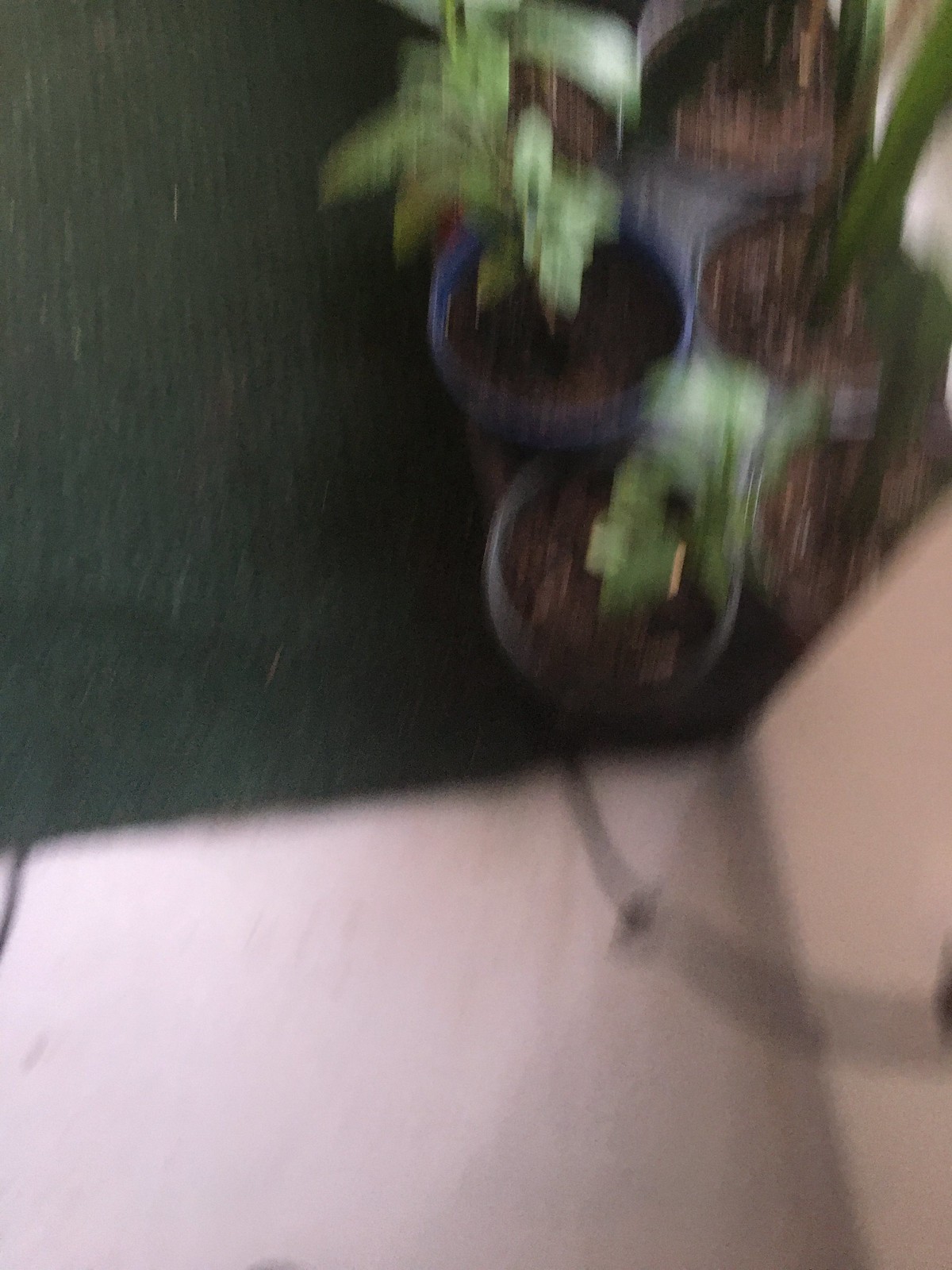In this blurry photograph, a number of circular black plastic pots containing green plants are arranged in vertical columns in the upper right corner of what appears to be a backyard area. The lower half of the image features a white surface extending upwards into a white wall. A blurry black line curves from the bottom right corner towards the group of pots. To the left, the surface transitions to dark green turf or grass, adding a touch of natural texture to the scene. Despite the blurriness, the vibrant green of the plants is discernible, providing a hint of life and growth within the image.